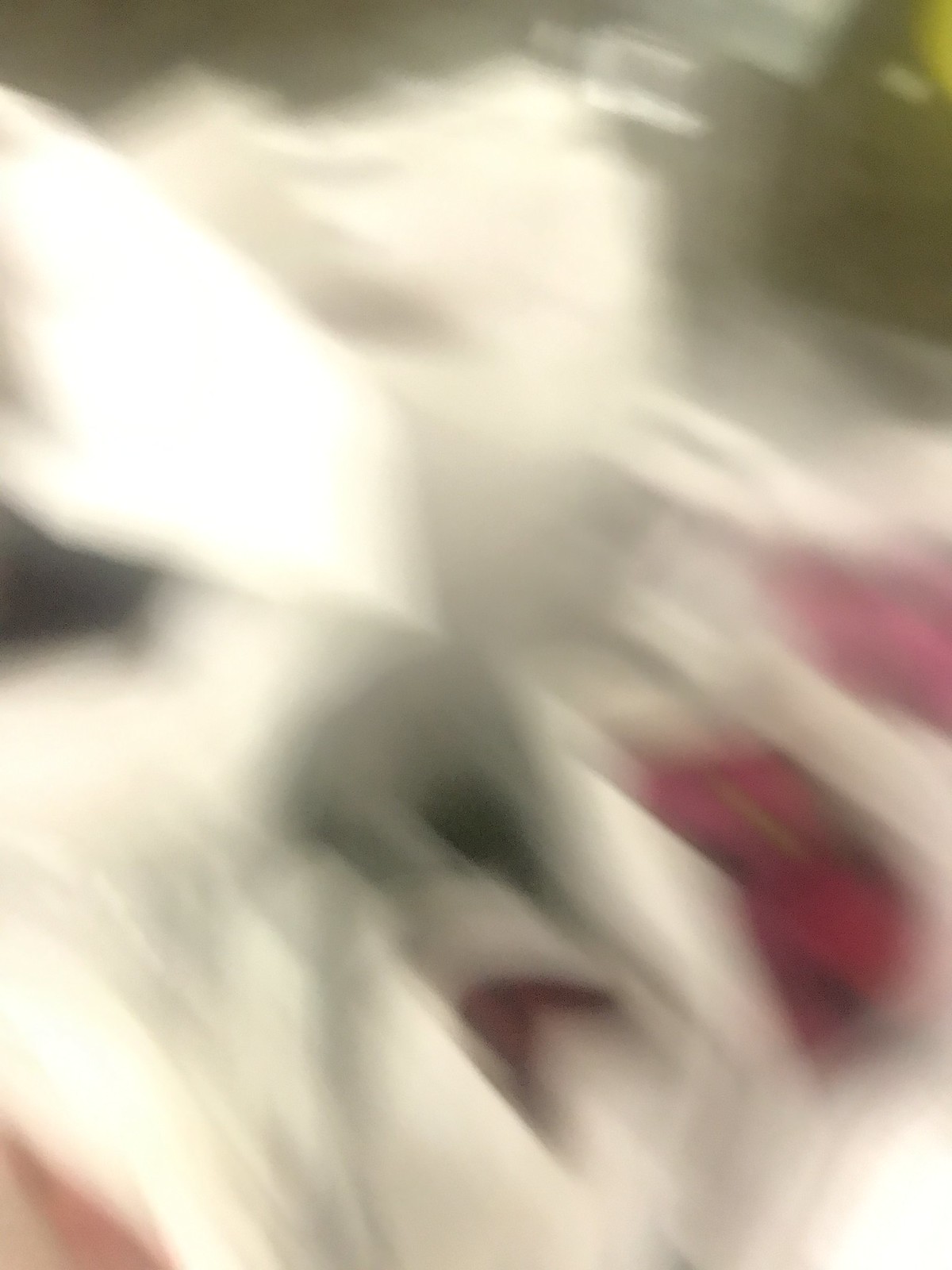This image is a very blurry and stretched photograph that makes it difficult to discern its subject matter. Predominantly, it features a lot of white shapes that resemble tall white plastic bags. Some of these bags appear to have red items inside, with noticeable reddish shadows towards the bottom right and left of the image. The top right corner has a yellowish hue, possibly indicating some light or another object with a yellow color. Additionally, there are hints of a green background, suggesting the photo might have been taken outside, potentially with green trees behind it. The image also contains some bone-like shapes or straight lines with rounded openings, evoking a vague resemblance to a skeleton viewed from above. Despite these observations, the overall blurriness and abstract nature of the image make it challenging to definitively identify its content.